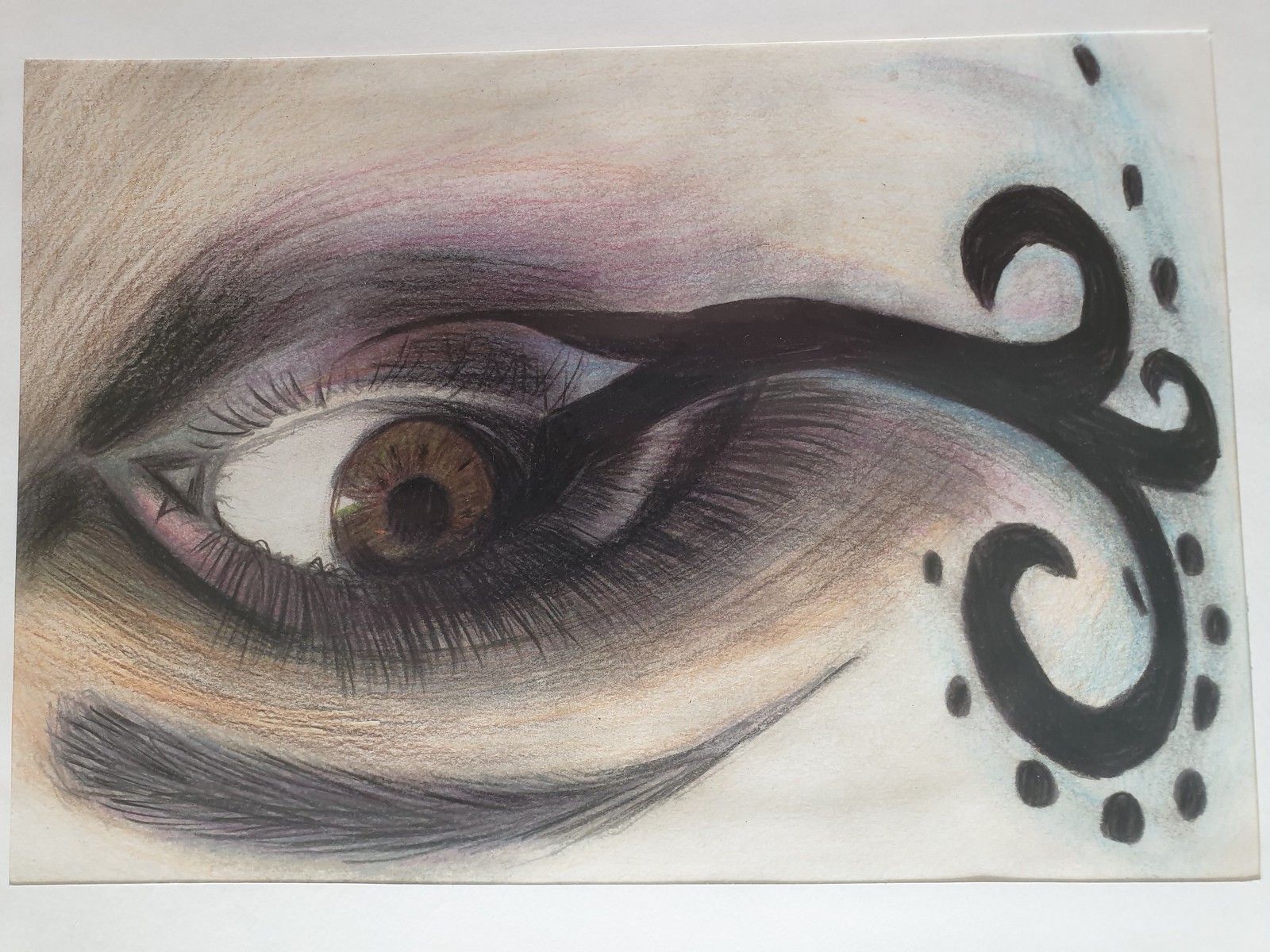An intricately detailed, colorful illustration is presented, albeit displayed upside down, on pristine white paper against an equally white background. The focal point of this artwork is a meticulously drawn brown right eye, gazing to the left. Above the eye, a thick, black brow adds depth and intensity. The eye is encircled with long, graceful eyelashes both on the upper and lower lids. Surrounding the eye is a dramatic dark purple shading, enhancing its vivid detail. Extending from the side of the eye is an elaborate design of a curving line, adorned with three distinct curves and dotted embellishments.